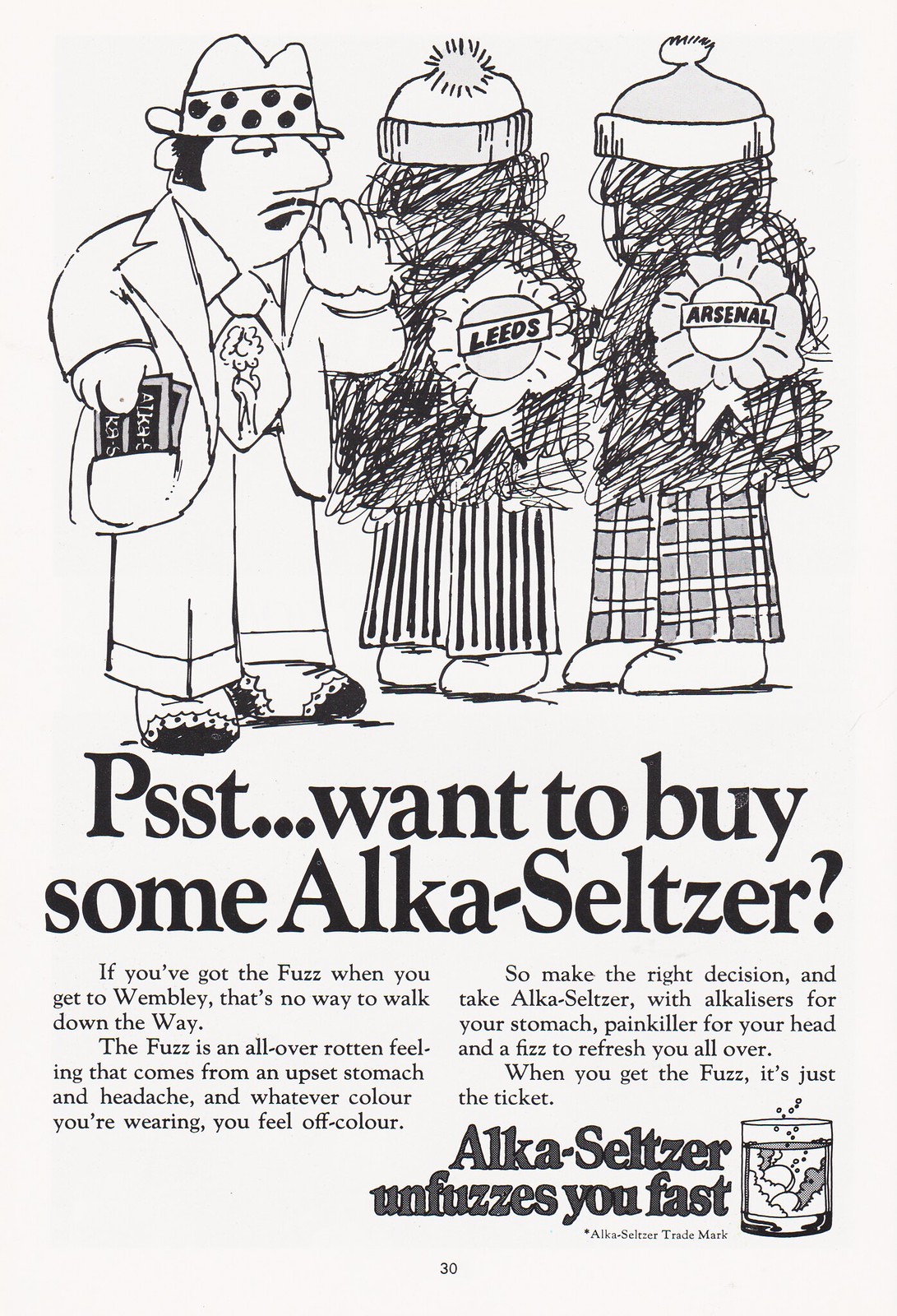In this black-and-white Alka-Seltzer advertisement, three cartoon characters are featured prominently. The central figure is a man in a suit with an oversized tie that features the image of a naked lady. He's depicted whispering conspiratorially, "Psst, want to buy some Alka-Seltzer?" while holding something that looks like individual packets of the product. He wears a distinctive mob hat with polka dots. The other two characters, labeled "Leeds" and "Arsenal," are mostly obscured by scribbles, but they are identifiable by their quirky attire, including striped or patterned pants and puffy hats.

The ad's narrative highlights the concept of "the fuzz," described as an all-over rotten feeling stemming from an upset stomach and headache. The main text explains, "If you got the fuzz when you get to Wembley, there's no way to walk down the way." It elaborates that feeling "off-color" can be remedied by using Alka-Seltzer, which combines alkalizers for the stomach, painkillers for headaches, and a fizz that refreshes you all over. The tagline underscores the product's efficacy: "Alka-Seltzer unfuzzes you fast."

At the bottom right of the ad, there's an image of a glass with a dissolving Alka-Seltzer tablet, reinforcing the product's promise to alleviate discomfort swiftly. The Alka-Seltzer trademark and the number "30" are also visible, contributing to the overall vintage feel of the advertisement.